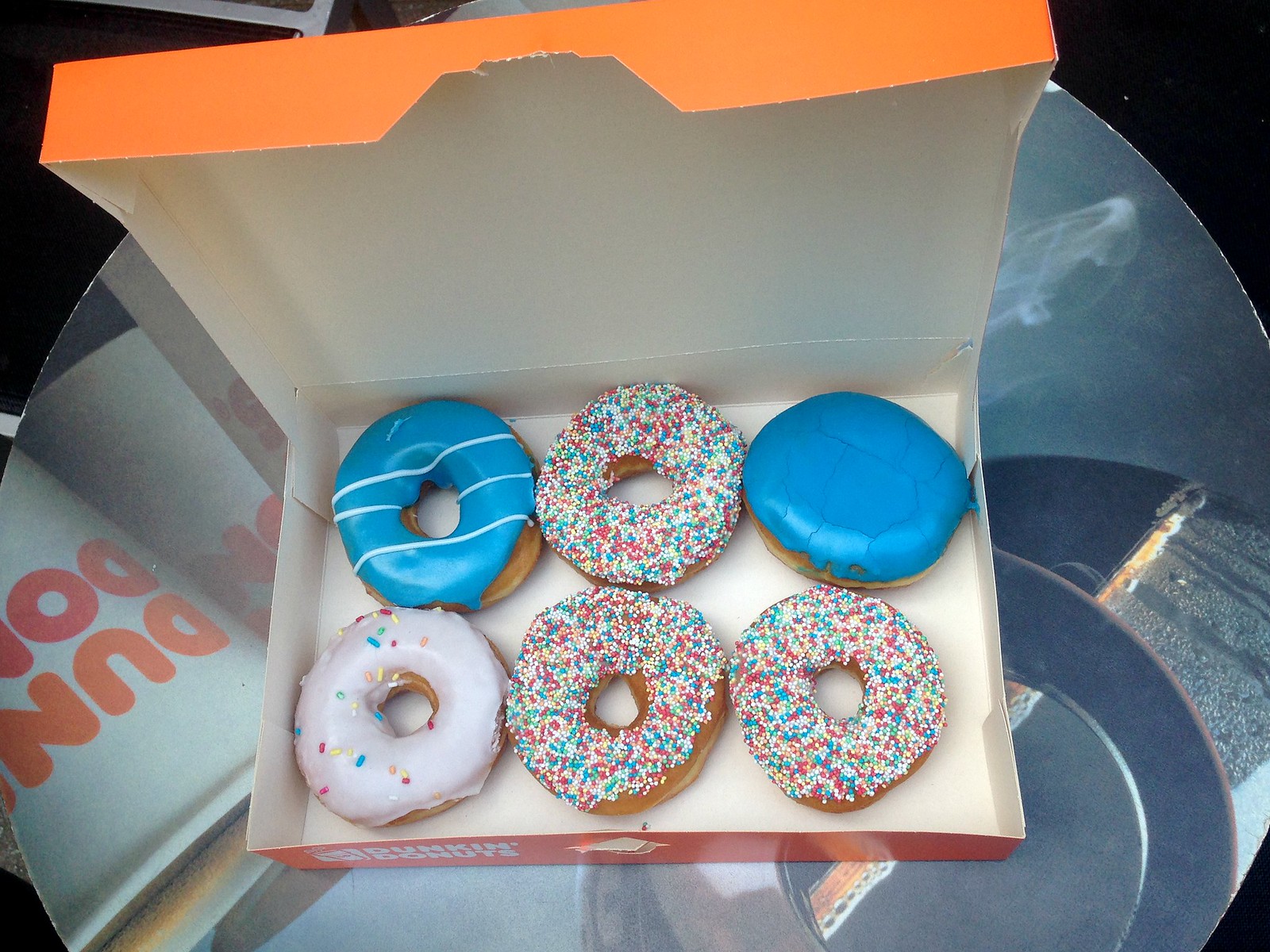In the image, a vibrant orange Dunkin' Donuts box is opened up inside a car, showcasing a delectable array of six donuts neatly arranged in two rows of three. The box is white on the inside, and although the Dunkin' Donuts branding isn’t fully visible, the letters “D-U-N” and “D-O-N” can be made out. Among the donuts, two are covered in a rich blue icing, with one featuring a white icing drizzle. The assortment includes three donuts with a generous amount of colorful sprinkles crowning their white icing, completely obscuring the surface. One of these sprinkled donuts appears to have inadvertently shared some of its decorations onto the adjacent donut with white icing and a sparse sprinkle coverage. The final donut stands out with its solid blue glaze and absence of a central hole, suggesting it might be filled with cream. To the left of the box, there is a sideways Dunkin' Donuts cup adding to the brand’s identifiable charm. The setting remains somewhat ambiguous, but it appears to be on a glass table within the vehicle.